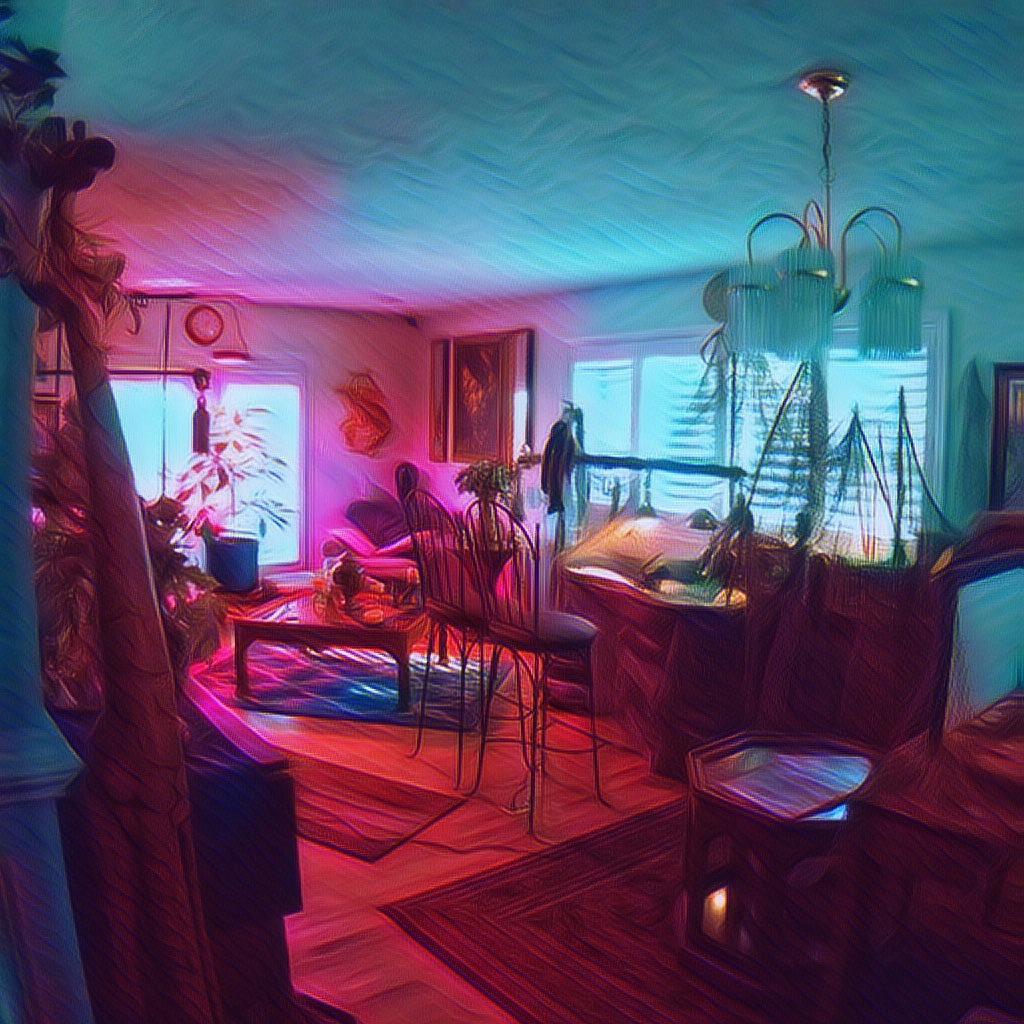The image presents an intricately stylized illustration of a living room bathed in a unique blend of pastel lighting, transitioning from pink on the left to blue on the right, giving it a dreamlike quality. On the left side of the room, there's a pair of double glass doors flanked by a pink tint, surrounded by various furnishings, including a dresser with a plant and a piece of clothing draped over it. A painting adorns the blue-tinged left wall, and above the doors, a clock with a brownish-red frame adds an antiquarian touch.

A chandelier with glass-like flutes and a gold band, suspended from a wire, hangs near the center, slightly offset from the bed positioned on the right. The bed, partially visible, hints at a more intimate setting with a bookshelf or another piece of furniture tucked behind it. Adjacent to the bed is a small dresser on a mat.

In the room's middle, a round coffee table on a blue rug faces two thin-framed, long-legged chairs with cushioned seats, positioned to look out a window embellished with blinds and netting. A longer runner rug complements the hardwood floor's warm tones further. Various artworks, potted flowers, and wall hangings contribute to the artistic ambiance, suggesting the living space of a creatively inclined individual.